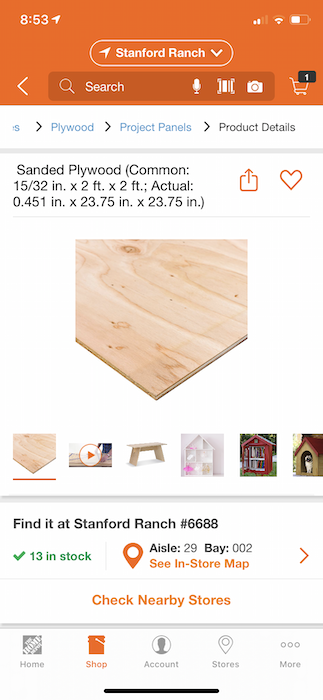The image captures a screenshot of a Home Depot mobile app interface at 8:53 AM. 

In the upper left corner, the time "8:53" is displayed, and on the right side, there are icons indicating cellular signal strength, Wi-Fi connectivity, and a half-full battery. The top center of the screen shows "Stanford Ranch." Below this line, there is a search bar containing a left-pointing arrow, a search field with the placeholder text "Search," a search icon, a microphone icon, a barcode icon, a camera icon, and a shopping cart icon displaying a notification with the number one.

Directly beneath the search bar is the product section, which notably displays the following text:

"S / Plywood / Project Panels / Details
Sanded Plywood (Common: 15/32 in. x 2 ft. x 2 ft.; Actual: 0.451 in. x 32.75 in. x 23.75 in.)"

To the right of this description are two orange outline icons: a square with an upward-pointing arrow and a heart. 

Below this text is a photo of the specified sanded plywood product. Under the photo, there is a row of six additional thumbnails related to the product.

An orange line separates this section from further details below:

"Find it at Stanford Ranch #6688
13 in stock
Aisle 29, Bay 002
See in-store map"

Following this is a right-pointing arrow and the text "Check nearby stores."